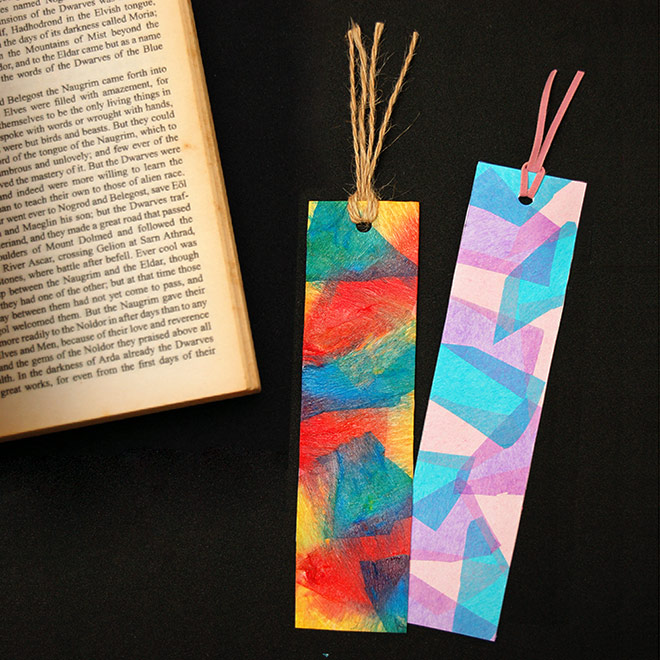The image features two vibrant and colorful bookmarks with abstract designs and a book page. The bookmark on the left has a teal triangle at the top with yellow, red, and blue shapes running down its front. It is adorned with light beige-colored yarn. The bookmark on the right showcases a light lavender and light turquoise surface, accented by a light pink ribbon at the top. It also has an abstract design with various shapes stacked on top of each other in blue, pink, and beige colors. The left side of the image includes a page from a book, which contains black, serif-style text and appears slightly aged with yellowed pages.